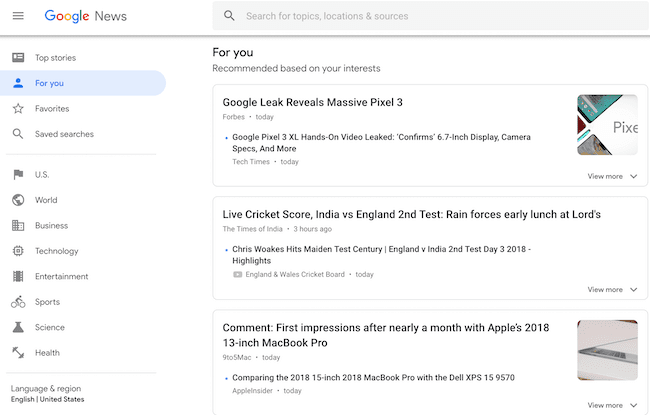A detailed caption for the described image:

The image showcases a computer screen displaying the Google News homepage. At the top of the page, "Google News" is prominently displayed in Google's signature multicolored letters. Directly beneath the heading, it reads "Top stories for you," with "for you" highlighted in blue, indicating the user has selected this section. 

On the left sidebar, various icons and corresponding labels are visible, including "Top stories for you," "Favorites," "Saved searches," "U.S.," "World," "Business," "Technology," "Entertainment," "Sports," "Science," "Health," and at the bottom, "Language and region" which is set to "English / United States."

At the very top of the page, there is a search bar with the placeholder text, "Search for topics, locations, and sources." 

In the main content area under the "for you" section, there are several recommended articles based on user interests. The articles listed include "Google leak reveals massive Pixel 3," "Live cricket score: India versus England second test," and "Comment: First impressions after nearly a month with Apple's 2018 MacBook Pro."